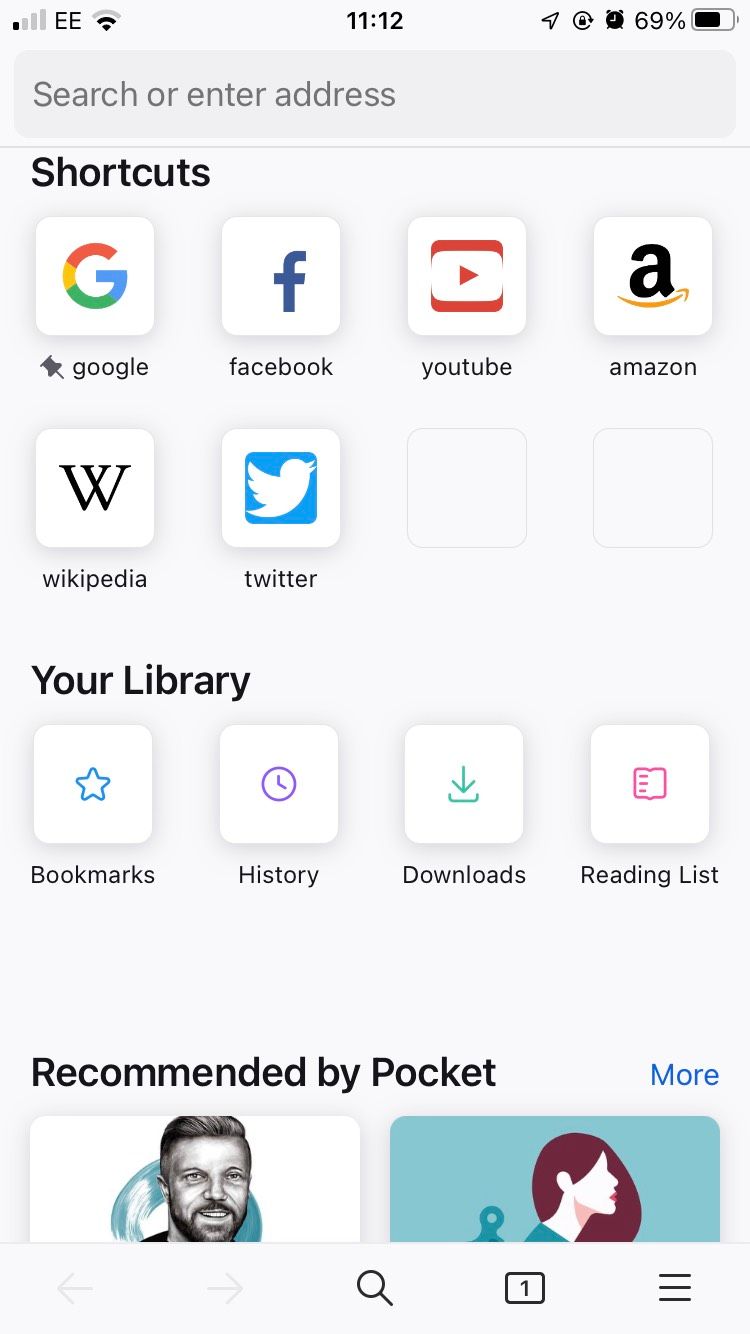This image captures a smartphone screen displaying a browser homepage with various shortcuts and status indicators. At the top left of the screen, you can see signal bars followed by "EE" and a Wi-Fi connectivity icon indicating network status. Centrally positioned, the time is displayed as "11:12" in black text. To the right, there are icons for airplane mode, refresh, a clock, and a battery icon showing 69% charge with a black line inside a white battery silhouette.

Below the status bar, the URL bar displays "Search or enter address." Underneath, there are several shortcut icons: Google, represented by a multicolored "G" with a pin icon; Facebook, shown as a white "F" inside a blue box; YouTube, identified by a red play button; Amazon, depicted with a capital "A" and an orange swoosh; Wikipedia, represented by a "W"; and Twitter, showcased by a small bird icon. Further down, sections for "Your Library" including bookmarks, history, downloads, and a reading list are visible. The bottom of the screen features a "Recommended by Pocket" section.